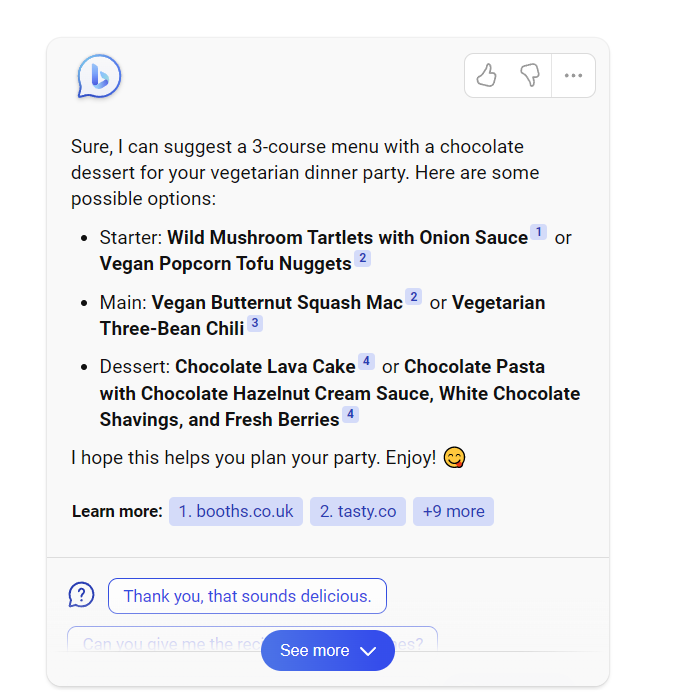**Detailed Caption:**

The image depicts a help chat interface displayed within a white square frame, accented by a light border. In the top corner, there is a lowercase letter “b” enclosed in a speech bubble. Adjacent to this, the menu features thumbs up and thumbs down icons, likely for user feedback. Below this section, a helpful suggestion is presented: "Sure, I can suggest a three-course menu with a chocolate dessert for your vegetarian dinner party. Here are some possible options."

The suggestions are organized with bold titles, starting with:

1. **Starter**: Choices include wild mushroom crostini with onion sauce or vegan popcorn tofu nuggets.
2. **Main**: Options are vegan butternut squash macaroni or vegetarian green bean chili.
3. **Dessert**: Selections feature chocolate lava cake or chocolate pasta with chocolate hazelnut cream sauce, white chocolate shavings, and fresh berries.

Following the menu, in regular print, is a cheerful note: “I hope this helps you plan your party and enjoy! 😊” with a smiley face emoji, tongue playfully sticking out.

At the bottom, two blue hyperlinked texts are provided for further reading: "boots.co.uk" and "tasty.co," with an additional option stating "plus nine more," indicating more links can be accessed. 

Finally, the user's response "Thank you, that sounds delicious," is shown, accompanied by an option to see more responses at the bottom.